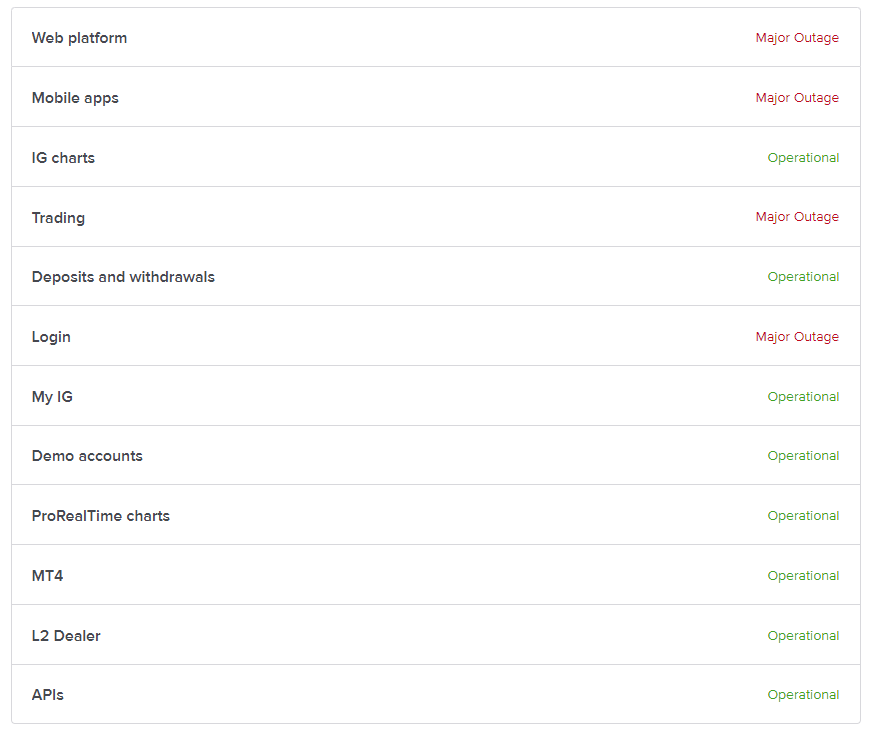A screenshot of the IG system status page displaying various services with their operational statuses. The page has a white background with a two-column, twelve-row table. The first column lists IG services including 'Web Platform', 'Mobile Apps', 'IG Charts', 'Trading', 'Pwns and Frauds', 'Login', 'My.IG', 'Demo Accounts', 'Pro Real Time Charts', 'MT4', 'L2 Dealer', and 'APIs'. The second column indicates the operational status of each service: 'Web Platform', 'Mobile Apps', 'Trading', and 'Login' are marked with "major outage" in bold red text, while 'IG Charts', 'Pwns and Frauds', 'My.IG', 'Demo Accounts', 'Pro Real Time Charts', 'MT4', 'L2 Dealer', and 'APIs' are marked "operational" in bold green text. The table is bordered by gray dividing lines on all sides, with additional gray lines separating each row and column. The arrangement of information is orderly, designed for quick readability regarding the system’s status.